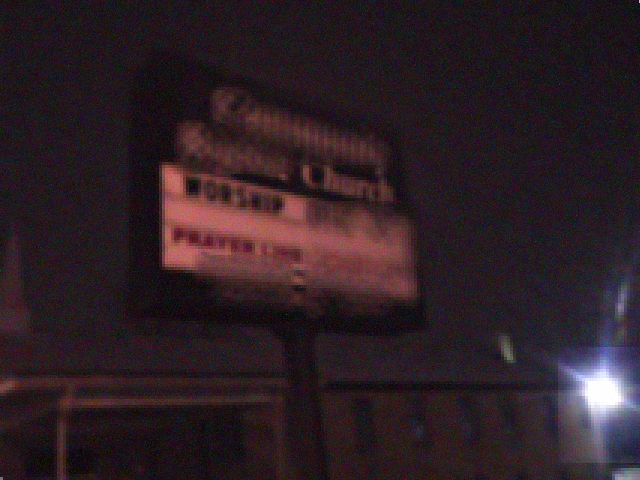This excessively blurry nighttime photo appears to be of a church sign, possibly taken from a backup camera, dash cam, or surveillance camera, given the deliberate blurring and a faint opaque rectangle overlay. Dominating the frame is a large, round post holding a square sign. The top half of the sign features a dark, almost black background with white letters; the third and only readable word is "church." The lower half of the sign consists of a white marquee section where letters can be manually placed. In this section, the word "worship" is clearly readable in black, and the word "prayer" is visible in red below it. The sign is situated in front of a building, likely the church itself, characterized by a brick facade, multiple windows, and an awning on its left. In the bottom right of the frame, a bright white light shines, contributing to the overall obscurity and hinting at the photo being possibly taken from a security device.